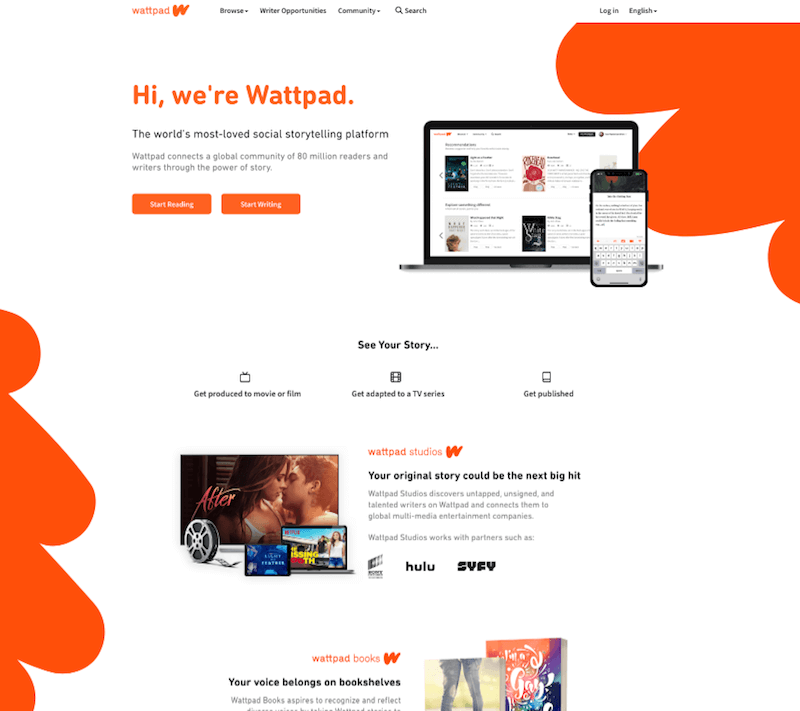Cropped Screenshot of Wattpad Product Website

This image is a detailed snapshot of the Wattpad product website, featuring a white background. 

At the top left corner, the Wattpad logo is prominently displayed. To the immediate right, there are three category options in small black font: "Browse" (with a drop-down menu), "Work Opportunities", and "Community" (also with a drop-down menu). Further right, there is a search bar, followed by the "Login" button and a language selection labeled "English" with a drop-down menu.

Below this, to the left, a large orange heading reads, "Hi, we're Wattpad". Beneath this, a subtitle describes Wattpad as "the world's most loved social storytelling platform," followed by a short descriptive text. Two prominent orange buttons are positioned underneath: "Start Reading" on the left and "Start Writing" on the right.

The top right section of the page displays an image of a laptop and a smartphone, both screens showing content akin to Wattpad pages. Additionally, an orange feathery graphic diagonally adorns the top right corner, while another orange graphic resembling fingertips is aligned vertically in the bottom left corner.

Centrally located on the page, the text "See Your Story" is featured, accompanied by three icons below it. These icons represent options for content creators: "Get Produced to Movie or Film" (with a TV icon), "Get Adapted to a TV Series" (center icon), and "Get Published" (third icon).

Below this section, a graphic on the left illustrates a computer screen with a movie title, a film reel, a tablet, and a laptop. On the right, the text promotes "Wattpad Studios" with the statement, "Your original story could be the next big hit," followed by a descriptive text. Three logo icons for Hulu, Syfy, and another film studio underscore the promotional content.

This comprehensive caption captures the essence and layout of the Wattpad product website as depicted in the cropped screenshot.